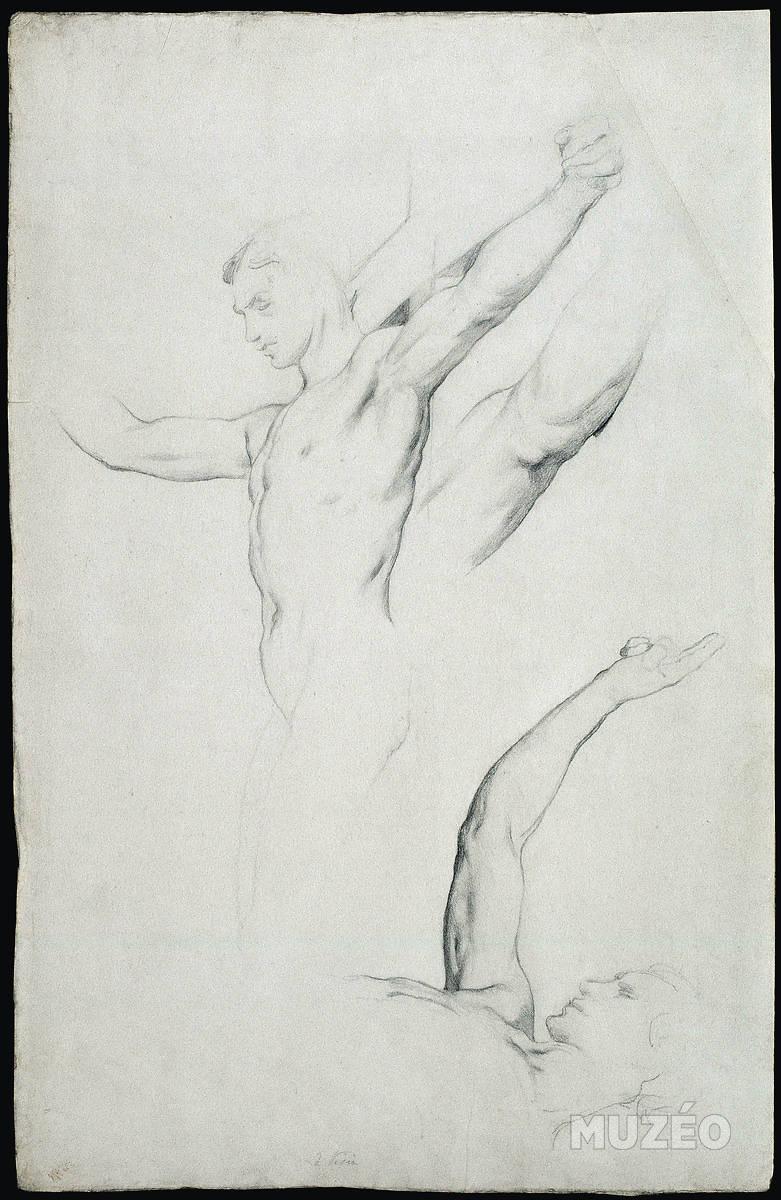The image is a detailed pencil sketch in black, white, and gray, vertically arranged on a tall piece of paper. Central to the drawing is a male human figure, depicted from the thighs up with a strong emphasis on the musculature and anatomy of the upper body. The figure is stretched out in a pose reminiscent of Jesus on the cross, viewed slightly from the side. The left arm extends outwards to the upper right part of the image, while the right arm reaches towards the left. The lower body appears faint and less detailed. To the top, there is significant focus on the torso, chest, and arms, with intricate detailing capturing the physical form. Additionally, there are separate studies of arm details and a head in the bottom right corner. The only text is the word "Museo," presumably the artist's signature, located in the bottom right corner of the drawing.